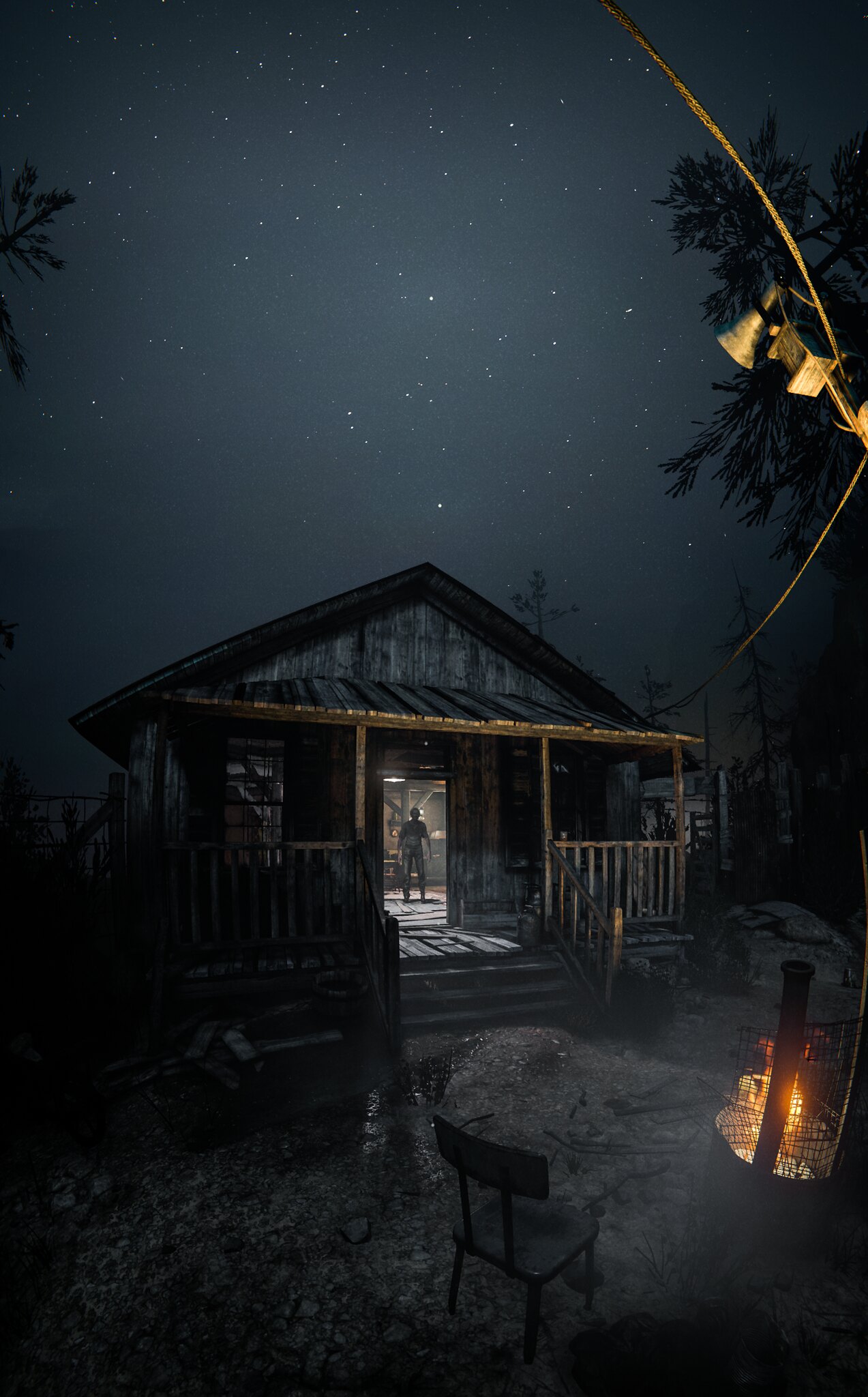In the middle of a dense wilderness, a small wooden cabin stands under a dark, starlit sky adorned with countless sparkling dots. The image, which has a painting-like quality, reveals the cabin's rustic features, including its modest porch. The scene is illuminated by a relatively small fire pit emanating from the bottom right corner. Near this fire pit, a single chair is placed, suggesting a spot for quiet contemplation. The ground around the cabin is visible, and leaves from a nearby tree frame the top edge of the image. Additionally, a golden hue graces the top right-hand corner, adding a subtle glow to the scene. The cabin's door is open, casting a warm light from within that contrasts with the dark surroundings. Standing in the doorway, a human figure casts a shadow, adding an element of mystery to the tranquil yet eerie nighttime setting.